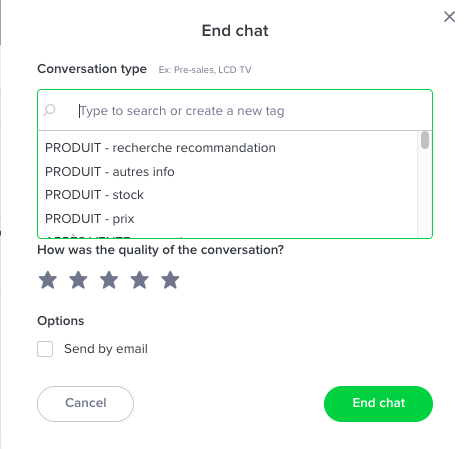The screen capture features an interface with a clean, white background and black and gray text, providing clear readability. At the top left, there is an option labeled "End Chat" next to a light gray 'X' icon. Below this, the interface specifies "Conversation Type," followed by the category "EX pre-sales LCD TV," enclosed in a thin green-bordered box. 

A white search field with a gray magnifying glass icon invites the user to "Type to search or create a new tag." Adjacent to the search field is a vertical gray scroll bar for navigation. 

Listed below "PRODUIT," the French word for "Product," are several categories including "PRODUIT Research Recommendation," "PRODUIT Autress Info," "PRODUIT Stock," and "PRODUIT Preaks," each in gray text. The last item is partially cut off. 

Beneath these categories is a section assessing conversation quality, represented by five gray stars. Further down, there is an "Options" section featuring a white box. 

At the bottom, two buttons appear: a gray-bordered "Cancel" button with an oval shape and a green, oval-shaped "End Chat" button with white text. To the side, there is a thin, vertical gray line.

The visual quality of the image is excellent, offering vision-impaired friendly design with no pixelation or blurring and no distractions from other images.